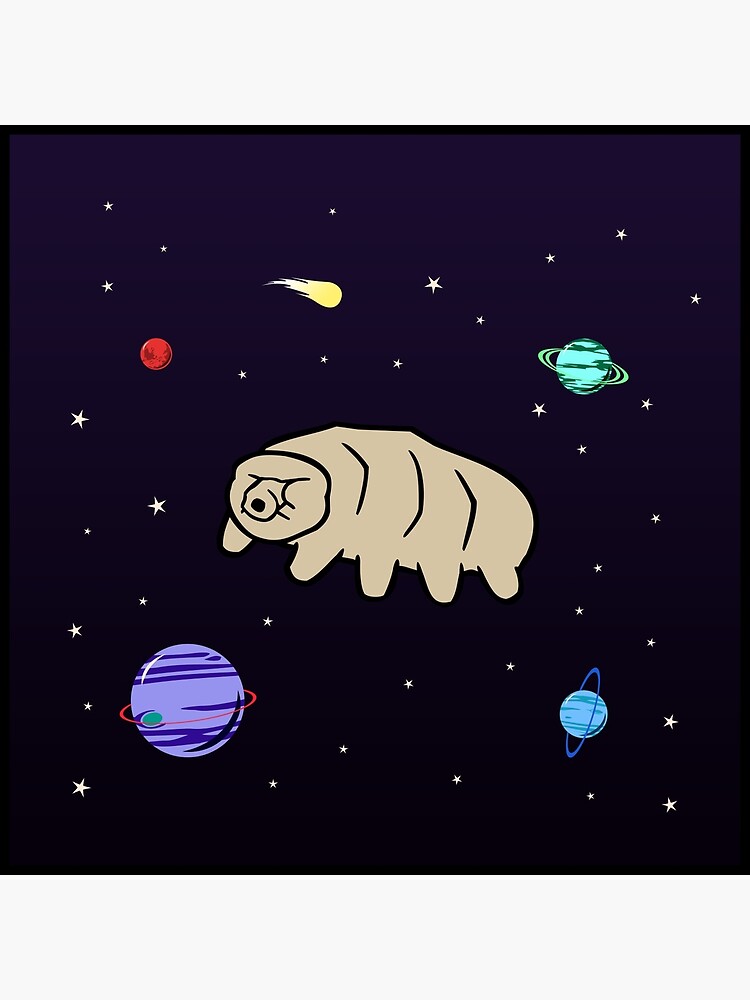This image depicts a whimsical, animated space scene set against a solid black background speckled with numerous white, five-pointed stars of various sizes. Dominating the center of the image is a grey tardigrade, a microscopic eight-legged creature resembling a plump caterpillar with a pig-like snout. Surrounding this cosmic traveler are several vividly colored planets, each adorned with rings, enhancing the outer space theme. 

In the lower right corner, there's a small planet encircled by a blue ring. The bottom left features a larger planet, primarily blue with a striking red ring. Above the tardigrade, on the upper left, lies a small red planet akin to Mars, next to a shooting star streaking across the sky. In the upper right, there's a blue planet with a green ring. The color-rich background and playful elements suggest the image might serve well as engaging, child-friendly artwork, suitable for nursery decor or youthful wallpapers. The detailed illustration, likely computer-generated, evokes a lighthearted and imaginative space adventure.